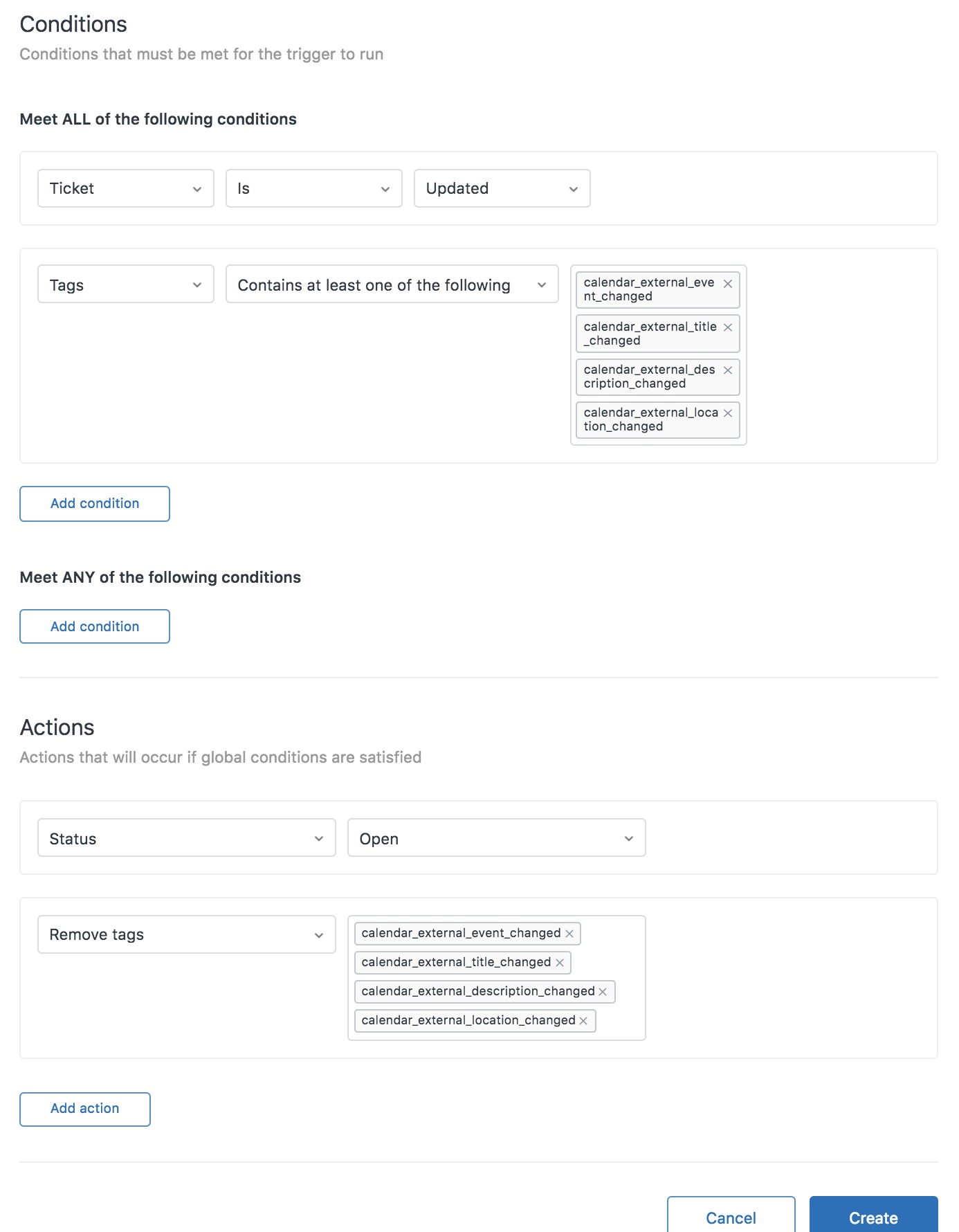This image depicts a detailed setup interface for configuring trigger conditions in a ticket management system. The interface is divided into several sections:

1. **Conditions to be Met for the Trigger to Run**:
   - **Ticket is Updated**: This is the initial condition that must be satisfied.
   - **Tags**: The next condition specifies that the ticket must contain at least one of the tags listed in the accompanying drop-down menu.

2. **Option to Add More Conditions**:
   - **Add Condition**: This button allows the user to add additional conditions that need to be met for the trigger to activate.

3. **Alternative Conditions**:
   - **Meet Any of the Following Conditions**: This section lets users specify alternative conditions that, if met, can also trigger the action. An "Add Condition" button is included here as well.

4. **Actions to be Taken if Conditions are Met**:
   - **Status Opened**: This action will set the status of the ticket to "Opened" once the global conditions are satisfied.
   - **Remove Tags**: This specifies that certain tags will be removed from the ticket.

5. **Configuration Options**:
   - Drop-down menus and buttons scattered throughout the interface provide customization options for each condition and action.

The image effectively showcases the granularity and customization possible within the system's trigger configuration tool.